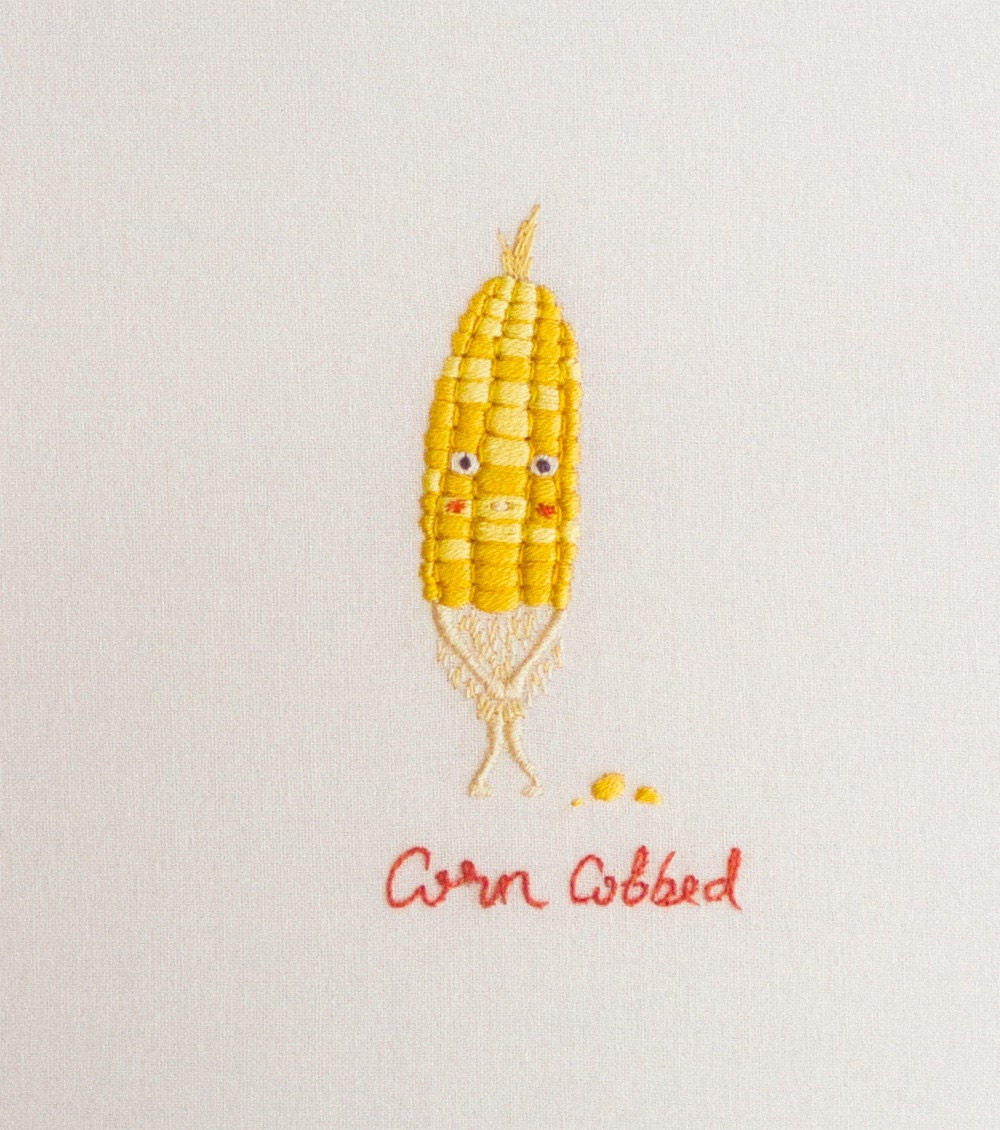The image showcases an intricately hand-stitched embroidery piece featuring a whimsical and shy corn on the cob. Positioned centrally on a textured white cloth background, the corn has its bottom half bitten off, giving it an exposed and bashful appearance. The corn character is depicted with far-apart eyes, a mouth, and red cheeks indicating embarrassment, while its arms attempt to cover the missing lower portion. Some kernels are scattered on the ground below it. The design is enhanced by various colors, predominantly yellow for the corn, with black, white, tan, and red accents. Beneath the central figure, the phrase "Corn Cobbled" is meticulously stitched in cursive thread. This charming and humorous piece, with its detailed stitching and playful elements, appears perfectly suited for display in a kitchen.